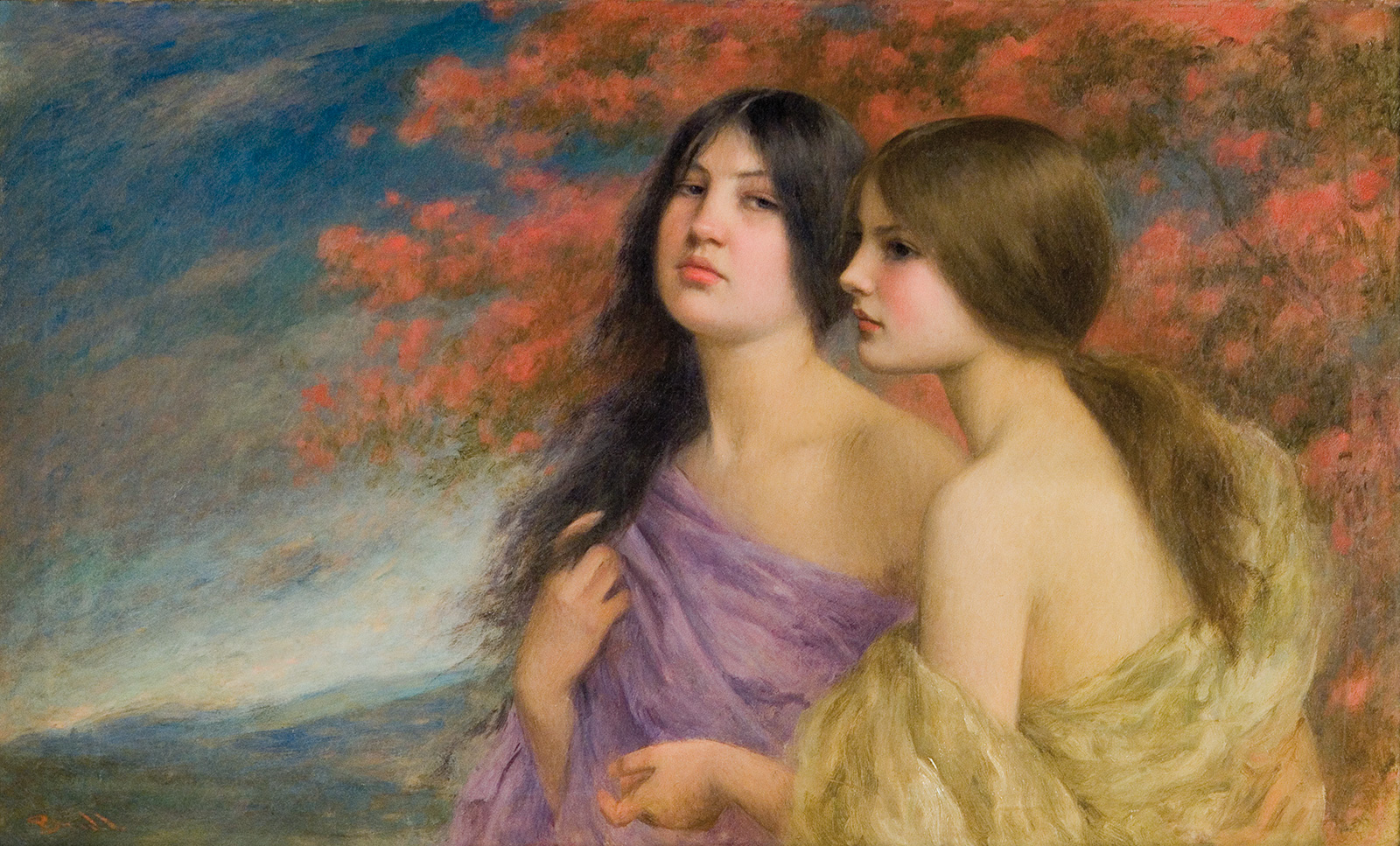The painting depicts two young women against a serene countryside background. The woman on the left, centrally positioned, gazes directly at the viewer with piercing dark eyes. She has long black hair flowing over her shoulders and wears a subtle, pinkish lipstick. Draped around her is a purple wrap, held up by her right hand, leaving one shoulder bare. Next to her, on the right, stands another woman with long brown hair adorned with rosy cheeks, also wearing similar pinkish lipstick. She is attired in a golden wrap that leaves her left shoulder and neck exposed, her profile view showing her contemplative gaze towards the left. The background complements the serene and intimate setting with a blue sky dotted with white clouds and rolling hills extending into the distance. Notably, a tree with striking pink and orange blossoms, reminiscent of a cherry blossom, adds a vibrant touch of color, enhancing the overall idyllic scenery.